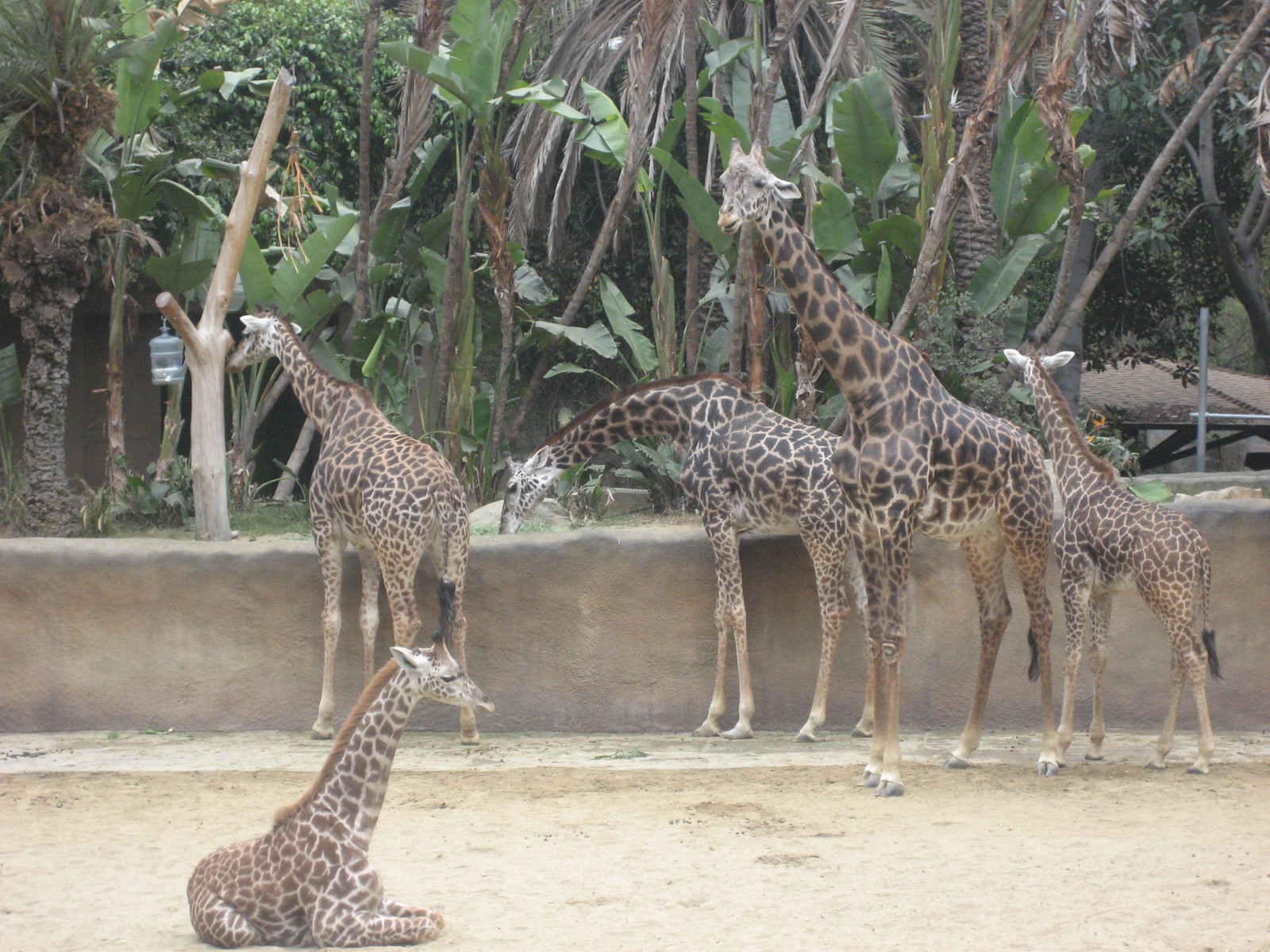In this zoo setting, the scene is dominated by a group of five giraffes, framed against a backdrop of tall, lush trees with big leaves, evoking a jungle atmosphere. In the foreground, a baby giraffe is sitting on its legs on a pale, dusty beige floor that looks like a mix of dirt and sand, typical of zoo enclosures. Behind this sitting giraffe, four others stand by a low, dirty brown stone wall, which they stretch their necks over as they graze and look around. The tallest giraffe is facing towards the camera, while another has its neck bent down, possibly eating. One giraffe appears to be inspecting a hanging container, potentially a water source, attached to a tree. The baby giraffe on the right is busy nibbling on some grass from a nearby bush. In the distance, the roof of a zoo building is visible on the right side, partially obscured by the verdant foliage and palm trees that populate the background.